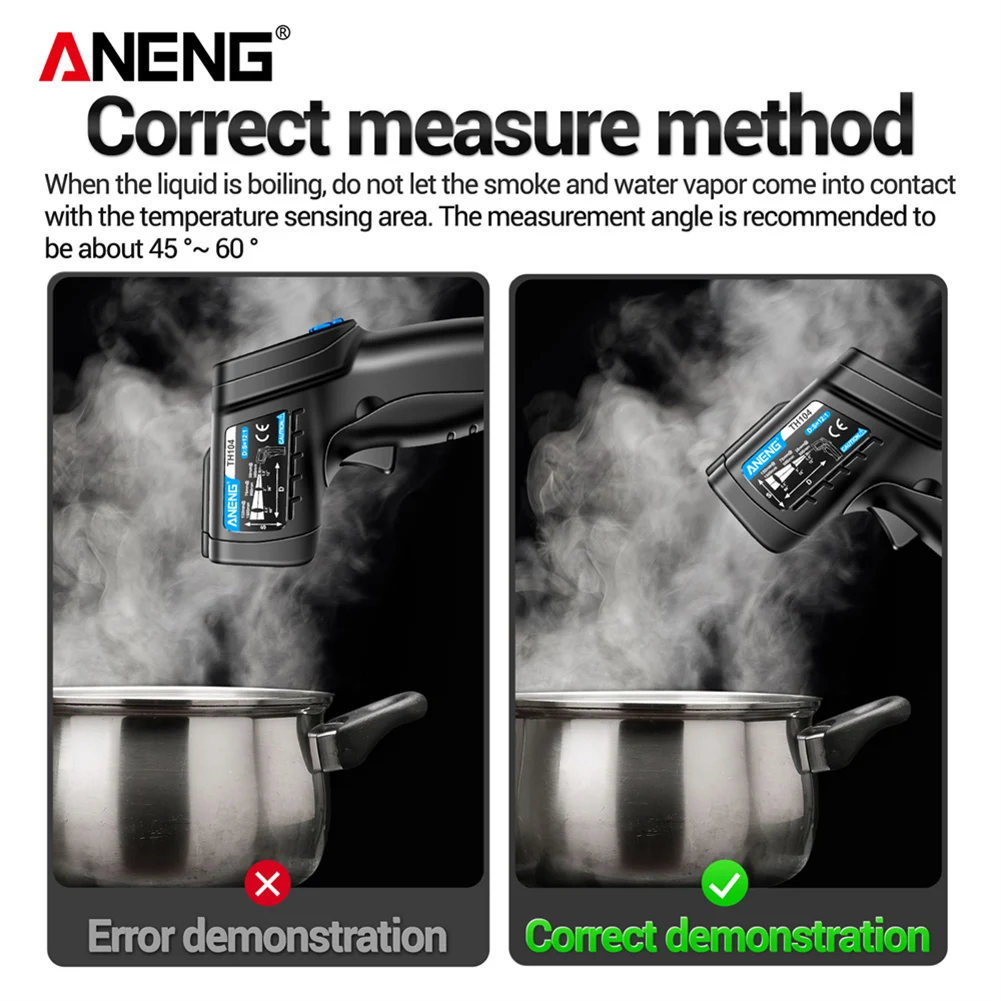The image is an advertisement for a temperature measurement device, likely a temperature gun, showcasing the correct and incorrect methods for measuring the temperature of boiling water. The top of the image is labeled "Correct Measure Method" and provides the instruction, "When the liquid is boiling, do not let the smoke and water vapor come into contact with the temperature sensing area." It also specifies that the recommended measurement angle should be between 45 and 60 degrees.

The left side of the image displays an "Error Demonstration" marked with a red circle and white X. It features a boiling, shiny silver pot with a black handle and large clouds of white steam rising from it. The temperature gun in this demonstration is pointed straight down into the water, which is indicated as incorrect. 

Meanwhile, the right side of the image shows the "Correct Demonstration," marked with a green circle and white check mark. Here, the same type of boiling pot is shown, but the temperature gun is angled diagonally toward the steam, adhering to the recommended measurement guidelines.

At the top left corner of the overall image, there is a triangular red logo followed by the letters "N, E, N, G" in capital letters. The setting is bright and clear, with ample lighting highlighting the clarity of the instructions and images.